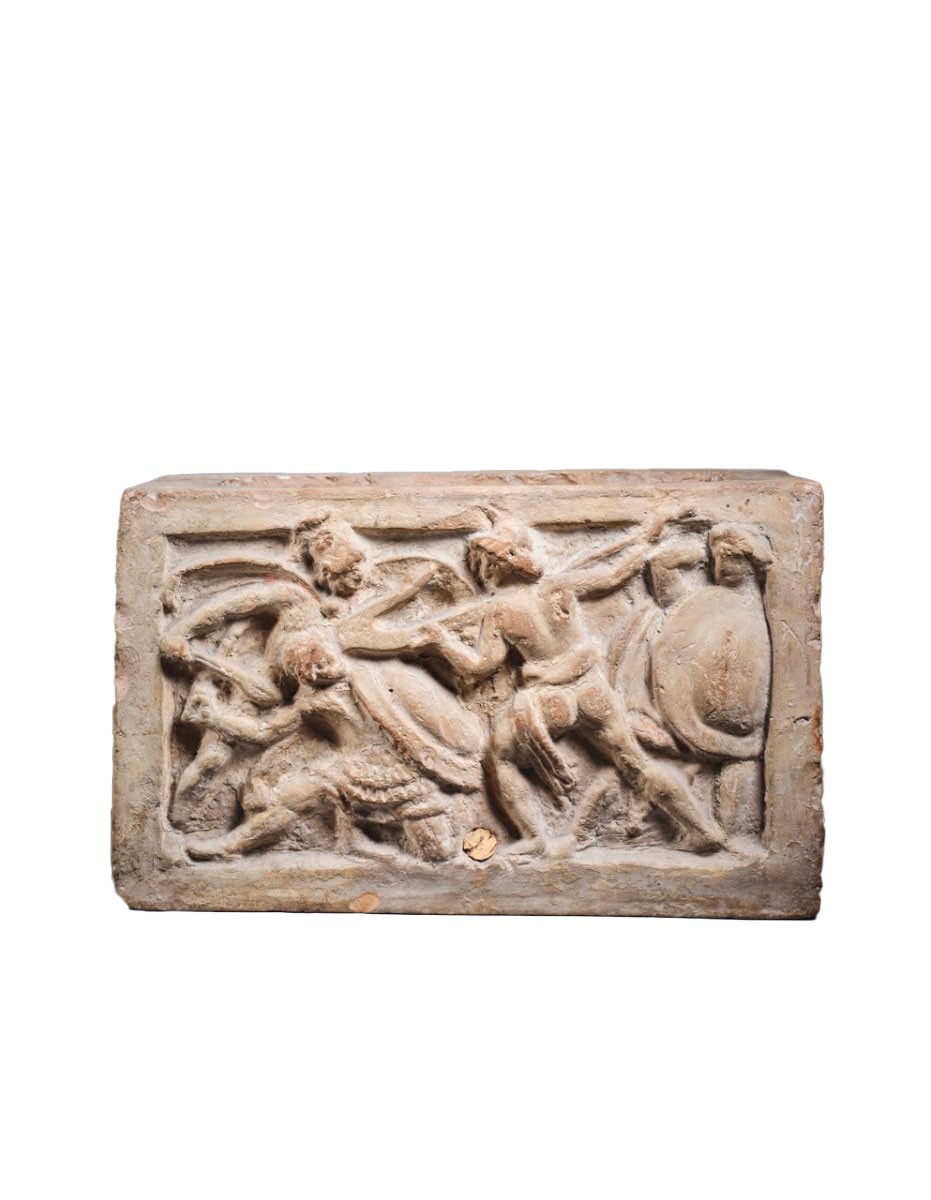This is a color photograph of a rectangular terracotta funerary urn from the 2nd century BC, depicting an ancient battle scene in raised relief. The urn, framed by a cracked and aged border, features several figures in dynamic poses against a white, isolated backdrop. Prominently, a soldier is preparing to throw a spear, positioned on his shoulder, while two other soldiers lean backward with shields in front of them. One figure is wearing a kilt-like garment that extends to his knees, and another wears a head garment with white around the waist. To the right, there is a partially indistinct figure or possibly an animal lying on the ground. The plaque displays a grayish hue with a tint of purple, adding to the historical and aged appearance of the artifact.